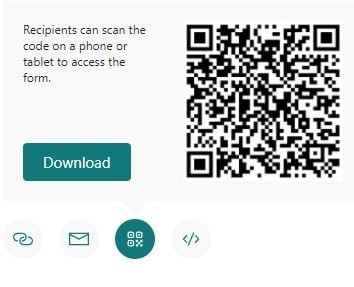This image features a white rectangular background with several interactive and informative elements. In the top left corner, there is a teal-colored rectangular button labeled "Download." Just above this button, a descriptive text instructs recipients to scan the adjacent QR code using a phone or tablet to access a specific form.

Dominating the right side of the image is a large QR code, occupying almost half of the page. This QR code includes distinctive black squares in its top two corners and the bottom left corner, typical of standard QR code designs.

Running diagonally from the bottom left to the top right, a dividing line separates the QR code section from the other graphics. Along the bottom of the image, there is an illustration of two interlinked circles, resembling a chain. Nearby, an envelope icon is depicted next to a blue circle containing four small pictures, and at the very bottom, there are two arrows pointing in opposite directions, one to the left and one to the right.

This minimalistic yet informative design aims to guide recipients efficiently on how to download and access the intended form by scanning the QR code.